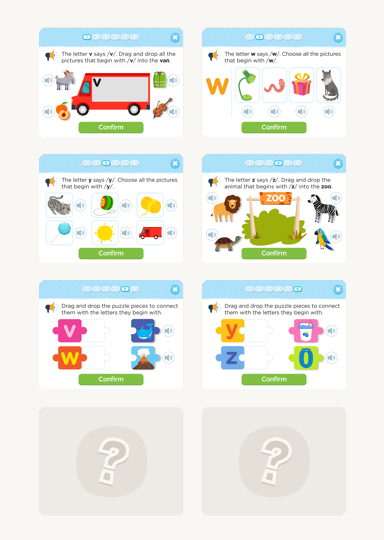The image resembles an educational card game designed for children, featuring a vibrant and interactive layout aimed at teaching phonics and letter recognition. The background is an almost white, very pale gray, set in portrait mode. There are eight horizontally oriented rectangles arranged in two columns and four rows.

- **Bottom Two Rectangles:** Light gray with a slightly darker gray circle and a thick, white outlined question mark in the center of each. These appear to be placeholders or hidden elements yet to be revealed.

- **Top Three Rows:**
  - Each rectangle in these rows has a light blue band at the top with white text and a close icon (X).
  - Beneath the blue band is a white background featuring colorful, child-like drawings and illustrations.

**Top Row:**
  - **Left Rectangle:** A red van with a "V" on it, alongside illustrations of a donkey, peaches, a vest, and a violin. A green confirm button is beneath these images, suggesting interaction to identify which items begin with the letter "V."
  - **Right Rectangle:** A lamp, worm, present, and wolf, associated with the letter "W." Small speaker icons next to each illustration hint at audio feedback, likely to pronounce the corresponding word.

**Second Row:**
  - **Left Rectangle:** Contains illustrations that are not clearly described but include six different images.
  - **Right Rectangle:** Highlights a zoo theme with images of a lion, turtle, zebra, and parrot.

**Third Row:**
  - **Left Rectangle:** Features puzzle pieces—one pink with the letter "V" and one orange with the letter "W." The images include a whale and a volcano, encouraging the matching of letters to corresponding images.
  - **Right Rectangle:** Contains similar puzzle pieces displaying the letters "Y" and "Z," paired with illustrations of a zero and what appears to be yogurt, though the exact image for "Y" is uncertain.

Overall, the image is an interactive, educational tool aimed at young learners, combining visual, auditory, and tactile elements to teach letters and associated sounds through engaging exercises.